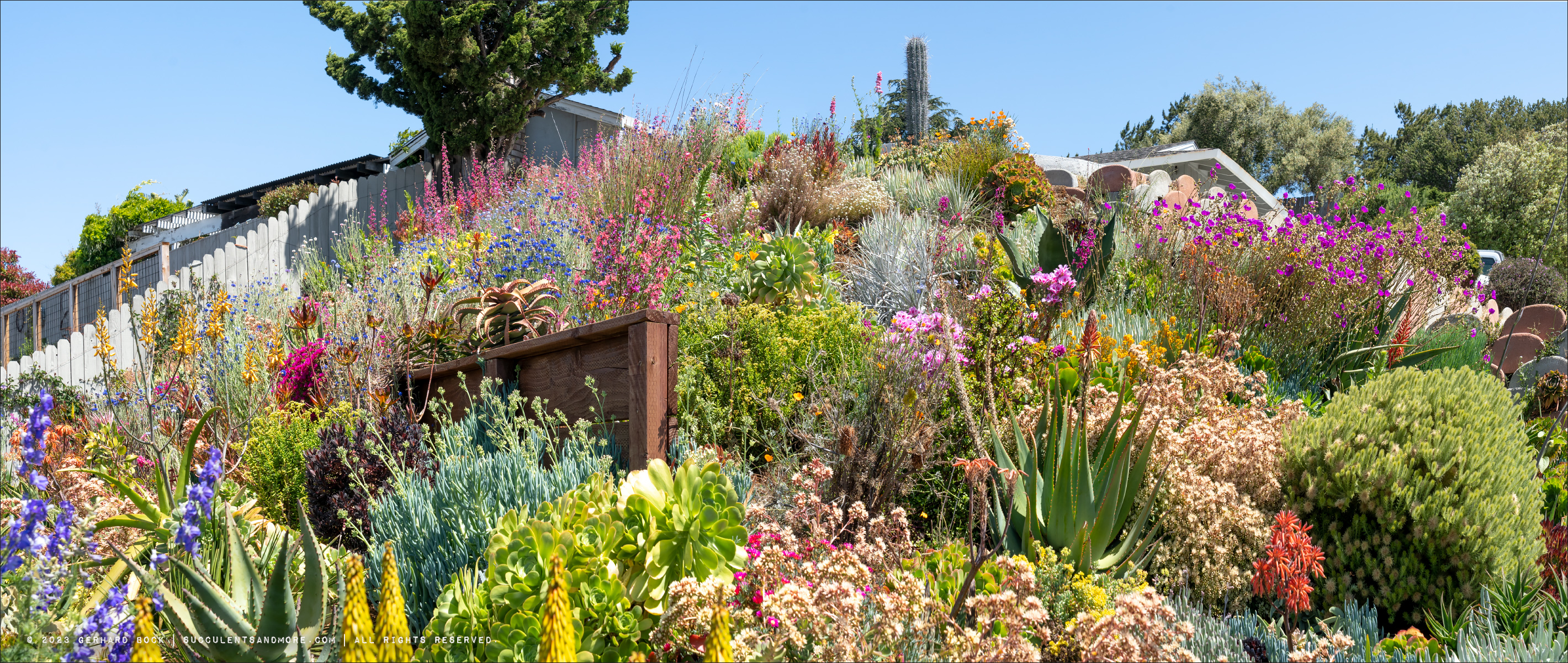The photograph captures a vibrant spring scene on a hillside adorned with a diverse array of flora. Bell-shaped flowers and cacti punctuate the landscape, their hues of red, purple, pink, yellow, orange, and green creating a colorful tapestry. Dominating the left side is a white picket fence climbing the hill, which is densely covered in plants and flowers. A large tree, slightly left of center, extends beyond the image's boundaries. A prominent cactus stands tall in the midsection of the frame, surrounded by a mix of bushes and smaller flowers. Toward the middle left, a brown sign is visible amidst the greenery. The upper portion of the image shows clear blue sky with no clouds, contrasting with the greenery below. In the distance, at the top of the hill, rooftops of residences peek out, suggesting a residential area beyond the floral slope. The overall setting is outdoors during daytime, with sunlight enhancing the vivid colors in the image.